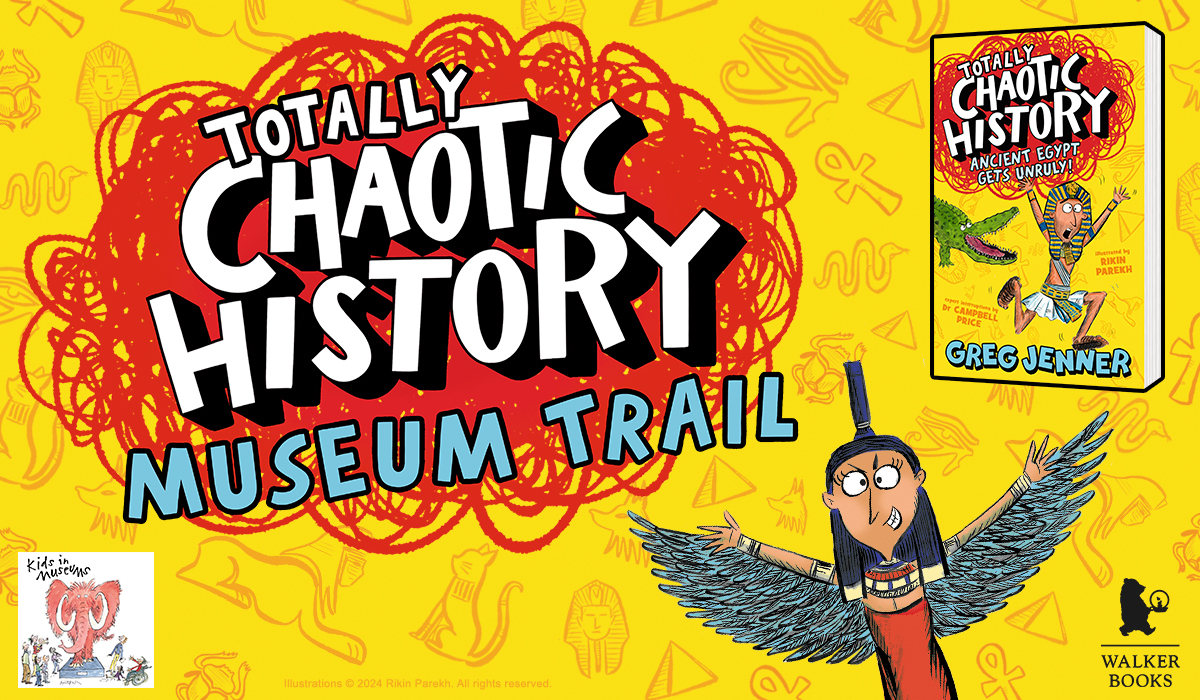The advertisement for the children's book "Totally Chaotic History: Museum Trail" by Greg Jenner features a vibrant, yellow background filled with various Egyptian-themed illustrations, including a Pharaoh's mask, pyramids, cats, eyes, snakes, and sphinx-like figures, suggestively hand-drawn. The main yellow background, decorated with orange hieroglyphics, further immerses viewers in an ancient Egyptian theme. In the upper right corner, an image of the book's cover shows a cartoon depiction of an Egyptian king running from a crocodile, with red scribbles and white text that reads "Totally Chaotic History" and blue text underneath that adds "Ancient Egypt Gets Unruly." This detailed imagery continues through the main banner, where a large red scribble on the left side contains the same white and blue text theme promoting the "Museum Trail." On the bottom right, there's a cartoon girl or woman in an ancient Egyptian outfit with feathered wings, positioned under the book cover thumbnail. The artist's name, Greg Jenner, is featured at the bottom in playful blue text, and the logo for Walker Books, depicting a bear, is placed in the bottom right corner. This colorful, chaotic design captures the essence of an adventurous journey through ancient Egyptian history.